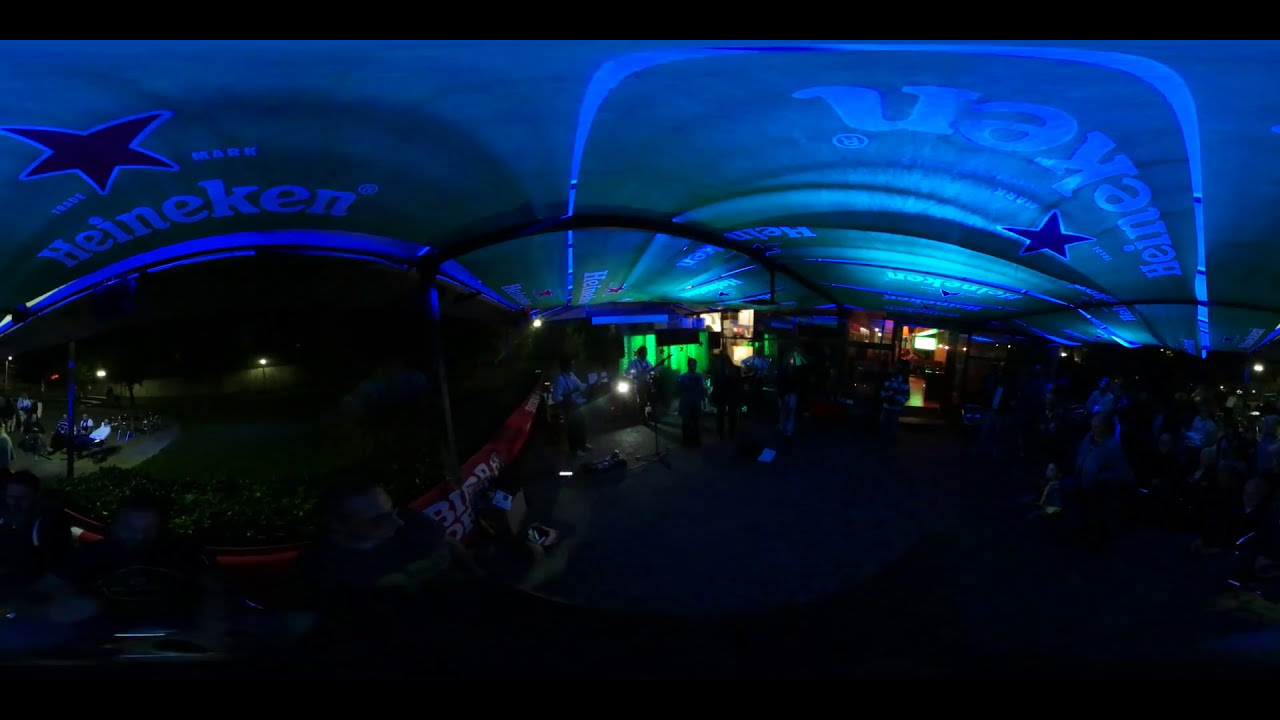The image captures a nighttime scene at an intimate concert venue, partially outdoors but under a dark green, Heineken-branded tent canopy. The ceiling prominently features the white Heineken logo and red star, with the text arranged in various orientations. The setting suggests a relaxed atmosphere with a bar-like venue vibe. The top third of the image is dominated by the Heineken tent, glowing subtly under low, orangish-yellow and green lights, contributing to the dim ambiance.

In the center of the image, under the tent, a band is playing, though the dim lighting makes the details hard to discern. To the left of the band, a red banner adds a splash of color, while various fans can be seen seated on chairs, enjoying the performance. The far left features an outdoor seating area with more individuals relaxing under the night sky, illuminated by street lamps. The overall scene evokes a calm, summer evening music festival sponsored by Heineken, with a decent crowd enjoying a laid-back concert experience.